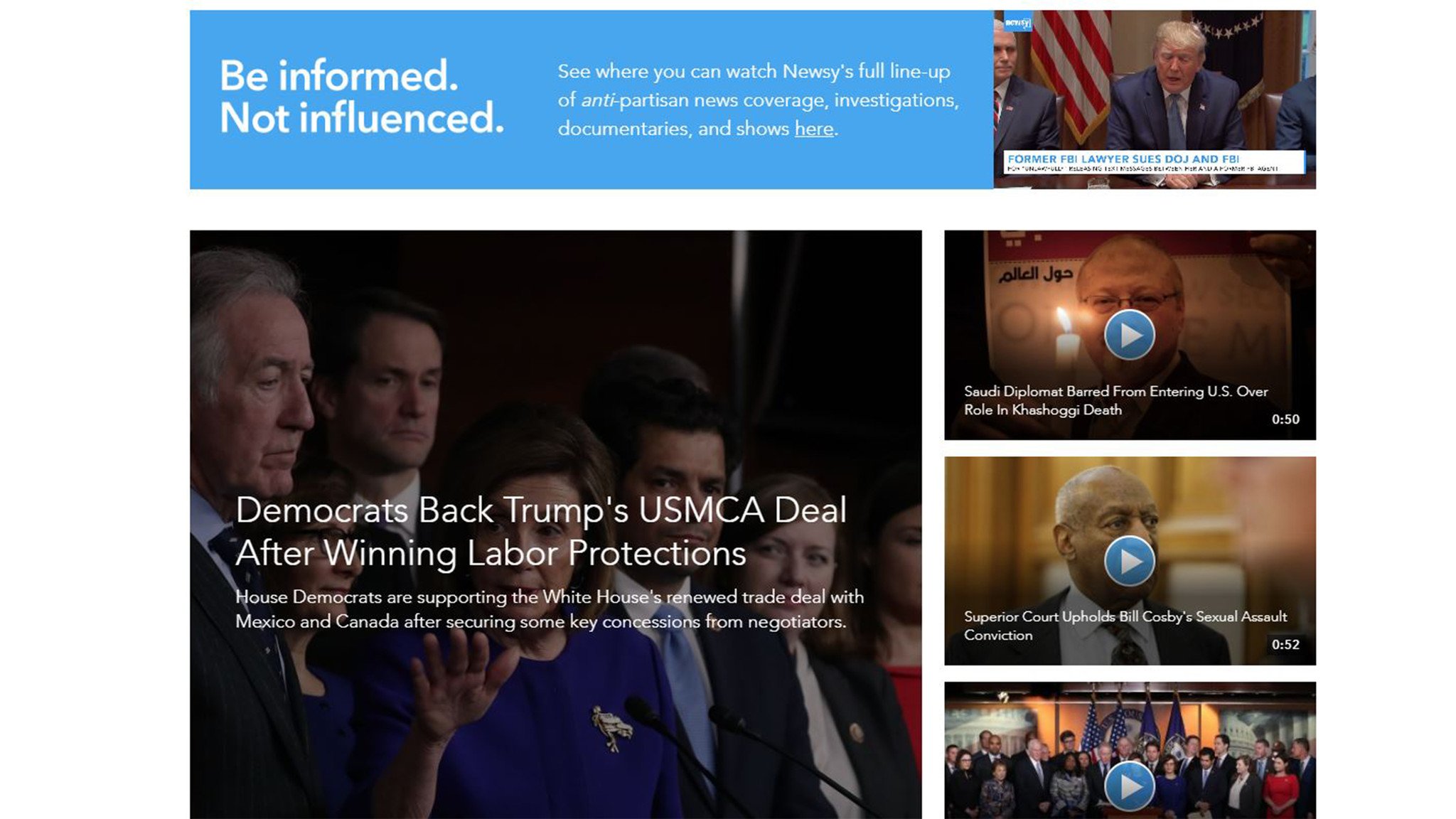**Caption:**

At the top of the image, a blue banner with white text reads: "Be Informed, Not Influenced." This banner promotes Newsy's comprehensive lineup of anti-partisan news coverage, including investigations, documentaries, and shows, with an interactive link for viewers to click and watch.

Lower on the image, a square panel headlines: "Democrats Back Trump's USMCA Deal After Winning Labor Protections." This section informs that House Democrats support the White House's renewed trade agreement with Mexico and Canada, achieved after securing essential concessions during negotiations.

In the top corner of the blue banner, a small square features a photo of Donald Trump alongside the text: "Former FBI Lawyer Sues DOJ and FBI." Adjacent to this, another clickable video title reads: "Diplomat Barred from Entering US Over Role in Khashoggi Death."

Further down, a text snippet informs that the "Superior Court Upholds Bill Cosby's Sexual Assault Conviction." The image also contains an additional, unrelated visual element without readable information.